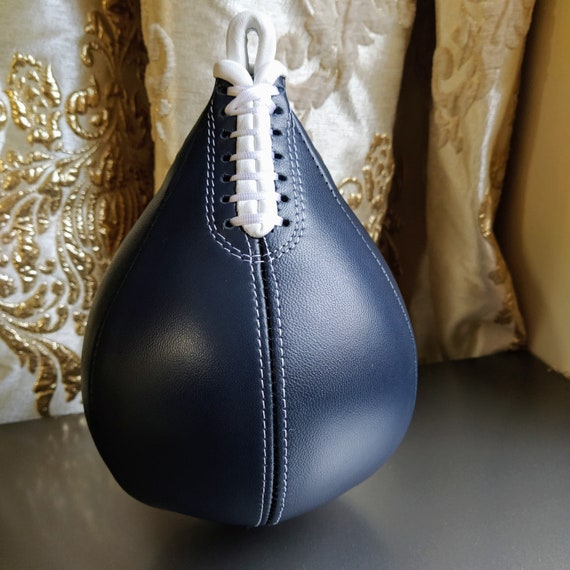This detailed color photograph features a small, navy blue leather boxing bag with a teardrop shape, prominently displayed on a reflective black table. The boxing bag, which appears brand new and unused, is adorned with white whip stitching and white laces at the top, which serves as a hanging mechanism. The stitching runs through the middle of the bag, showcasing both double and single threads in the design. 

In the background, there is a lush Baroque-style fabric draped in soft folds, likely staged by a window to accentuate the interplay of light. The fabric, satin in appearance, is a medium to light beige hue, embellished with dark golden swirls, fleur-de-lis motifs, and white embroidered patterns, giving it a rich, decorative look. This ornate backdrop adds an elegant contrast to the simple, modern design of the punching bag, creating a visually striking composition without any human or animal presence.